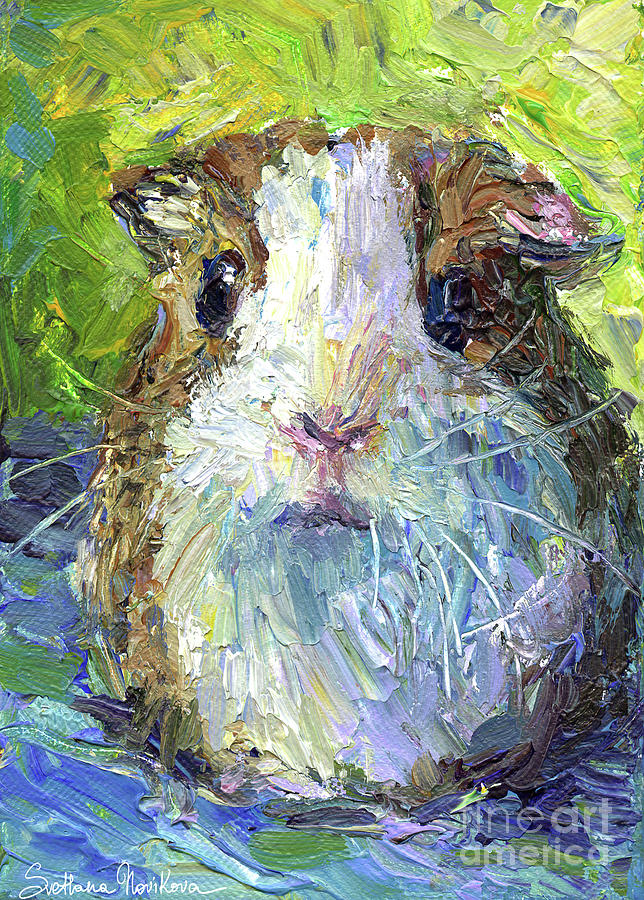This painting is an abstract, impressionistic depiction of a rodent, likely a hamster, rendered with minimalistic yet evocative brushstrokes. The creature features small ears, large expressive brown eyes, and a delicate white face adorned with whiskers and a pink nose. The background showcases a vibrant blend of greens and yellows, creating a dynamic and lively backdrop. In the foreground, the hamster appears to recline on a bed of broad blue and purple brushstrokes, reminiscent of the vibrant style characteristic of Van Gogh. The overall composition eschews realism in favor of an impressionistic approach, with colors seamlessly blending into one another to evoke a sense of whimsy and movement. The bottom left corner of the painting bears the signature of the artist, "A. Novikova," while the lower right corner includes a watermark from "Fine Art America."